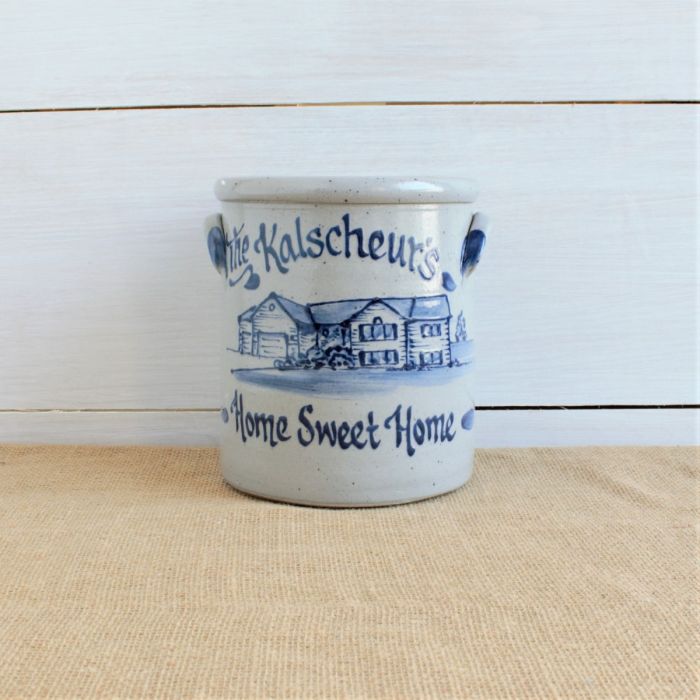In the image, there is a white ceramic canister, cylindrical in shape, resting on a brown, textured burlap material. The canister, adorned with dark speckles, features two small, close-to-the-body handles on either side. The centerpiece of the design is a detailed blue illustration of a charming two-story family house with a double garage and bushes in front. Above the illustration, in a script handwriting font, is the text "The Kalscheurs," with an apostrophe before the final "S." Below the house, the phrase "Home Sweet Home" is inscribed, also in blue. The canister, which looks suitable for storing kitchen items like flour or utensils, is placed centrally in the image, set against a backdrop of horizontal white wood boards evocative of shiplap, contributing to a cozy, homely aesthetic.